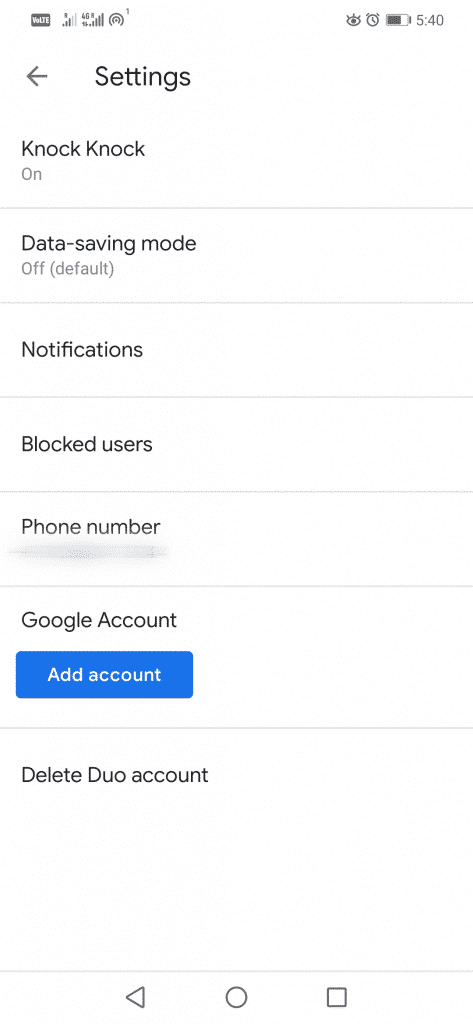The image captures the screen of a mobile phone displaying a settings menu. At the top of the screen, various status icons are visible, including a settings cogwheel, an eyeball, a clock, and a battery icon showing approximately 75% charge. The time displayed is 5:40. An arrow pointing left is labeled "Settings."

Directly below, the settings header reads "Knock Knock," indicated in bold black text, with "On" shown in grey. A faint grey line separates this from the next section labeled "Data Saving Mode," which is turned "Off" by default, also noted in grey text and parentheses.

Further down, another faint grey line divides sections. "Notifications" is written in bold black text followed by yet another grey separator. Below, "Blocked Users" is listed in bold black text with a subsequent grey line.

Next, "Phone Number" appears on the screen, but the text seems obscured with smudges, indicating possible deletion or erasure. A grey separator follows this section too.

Below that, "Google Account" is listed, accompanied by a blue rectangular button labeled "Add Account." The subsequent screen division continues with a grey line separating the final option, "Delete Dual Account."

At the very bottom of the screen, the navigation icons of a triangle, a circle, and a square are present, indicating options to go back, return to the home screen, or access recent apps.